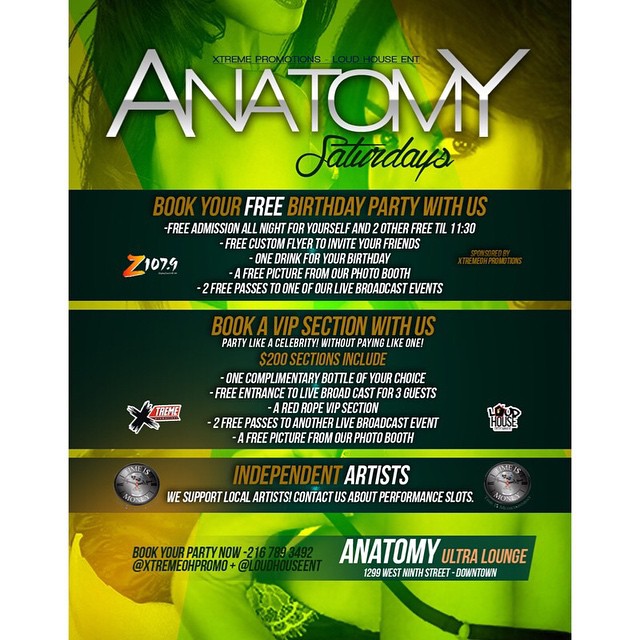This promotional flyer for Anatomy Ultra Lounge in Cleveland, Ohio, uses a striking blend of graphic design and a screened color photograph in yellow and green tones. Against this visually dynamic background, featuring two young women in low-cut dresses partially obscured by a green filter, the flyer prominently features the club's logo at the top in a white and gray gradient, with "Saturdays" written in bold black script.

The flyer, produced by Extreme Promotions and Loud House ENT, invites patrons to book a free birthday party, with enticing benefits like free admission for themselves and two guests until 11:30 PM, a custom flyer, one complimentary drink, a photo booth picture, and two free passes to a live broadcast event. The Z107.9 logo marks this section.

Further down, a dark green strip promotes booking a VIP section, promising a celebrity experience for $200. This includes one complimentary bottle, VIP entrance for three guests, a red rope VIP area, two passes to another live event, and a photo booth picture. This section features logos, presumably related to other promotional partners.

The flyer also champions local talent by inviting independent artists to contact them about performance slots, reinforcing the venue's support for the local art scene.

Concluding with key details, the flyer lists contact information and social media handles (@XtremeOHPROMO and @LoudHouseENT) and the lounge's address: Anatomy Ultra Lounge, 1299 West 9th Street, downtown Cleveland, Ohio.